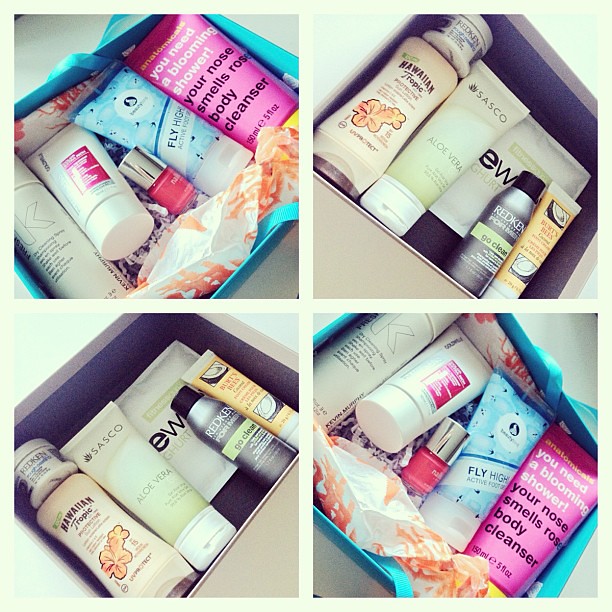This image is divided into four sections, each presenting a box of personal care and beauty products, arranged in a windowpane-style format. The upper left and lower right sections feature a blue basket filled with various items, including a pink and yellow tube of body cleanser labeled "you need a blooming shower, your nose smells rosy," a blue tube of "Fly High" active cream, red nail polish, a bottle with the letter "K," and another white tube with a pink logo. Both sections show the same contents but at different angles. The upper right and lower left sections display another set of personal care products, including a green and white tube of Sasko Aloe Vera, a tube of Hawaiian Tropic, a grey bottle of Redken for Men, and some Burt's Bees products. These two sections also mirror each other from different perspectives. The entire image showcases a colorful assortment of beauty products, emphasizing hues of pink, yellow, blue, green, and red across the various items.